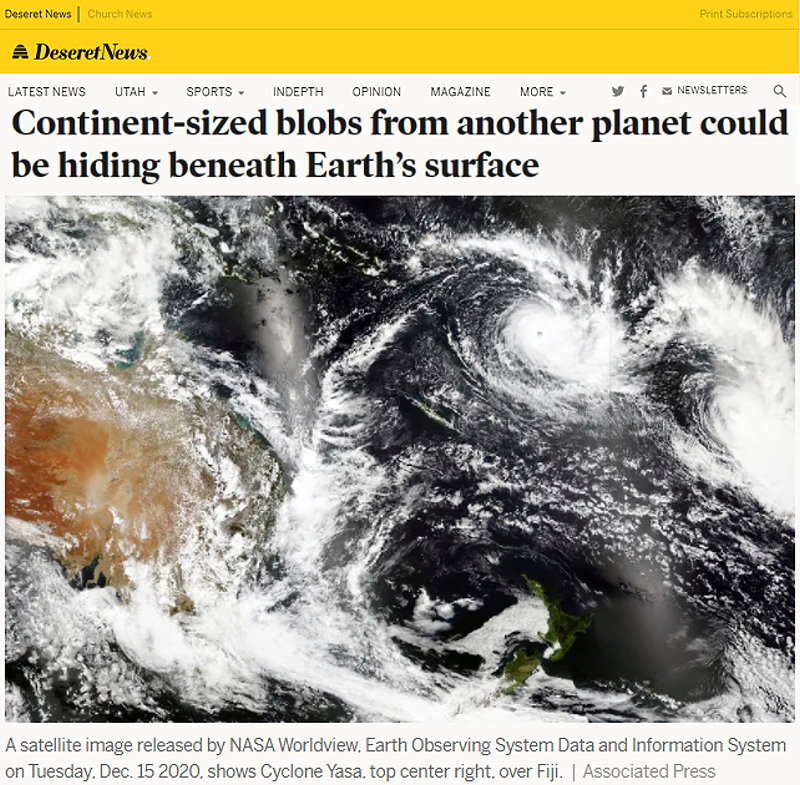This web page from Deseret News is distinguished by a gold banner at the top, prominently displaying "Deseret News" in black text in the left corner. Below, a white navigation bar contains various sections, including "Latest News," "Utah," "Sports," "In-Depth," "Opinion," "Magazine," and a "More" drop-down menu. The page also features social media icons allowing users to connect with Deseret News via X, Facebook, Email, Newsletters, and includes a search icon for browsing the site.

The focal point of the page is an article titled in bold black text, "Continent-Sized Blobs from Another Planet Could Be Hiding Beneath Earth's Surface." Accompanying the article is a satellite image showing hurricane activity. The image captures Cyclone Yassa situated at the top center-right over Fiji, as released by NASA's Worldwide Earth Observing System Data and Information System on Tuesday, December 15, 2020. The image credit is attributed to the Associated Press.